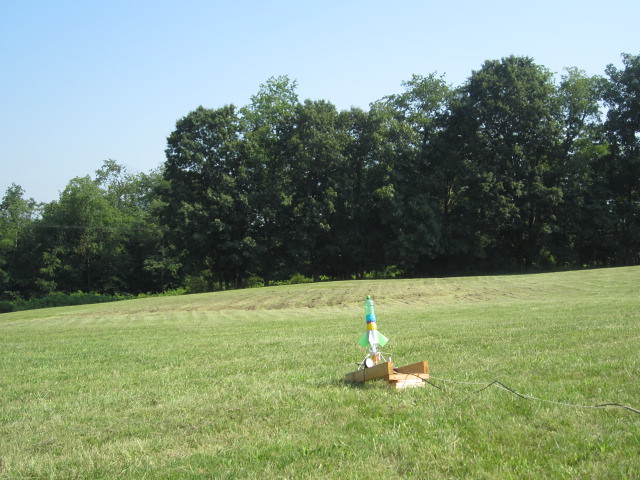The image depicts an outdoor setting in a lush green field, recently mowed, under a bright and clear blue sky. The background features a row of tall, leafy trees, adding depth to the scene. The focal point of the image is an improvised science project in the form of a small, colorful rocket made from a soda bottle. This bottle, green with a green lid, is mounted on top of a wooden launch pad. The rocket stands about a foot tall and is adorned with bands of various colors—yellow, purple, and blue—towards its middle. It features four light green wings at the base. Two wires, black and white, are attached to the rocket, likely for the launch mechanism. The overall scene suggests the anticipation of launching this homemade rocket into the sky on a bright, sunny day.